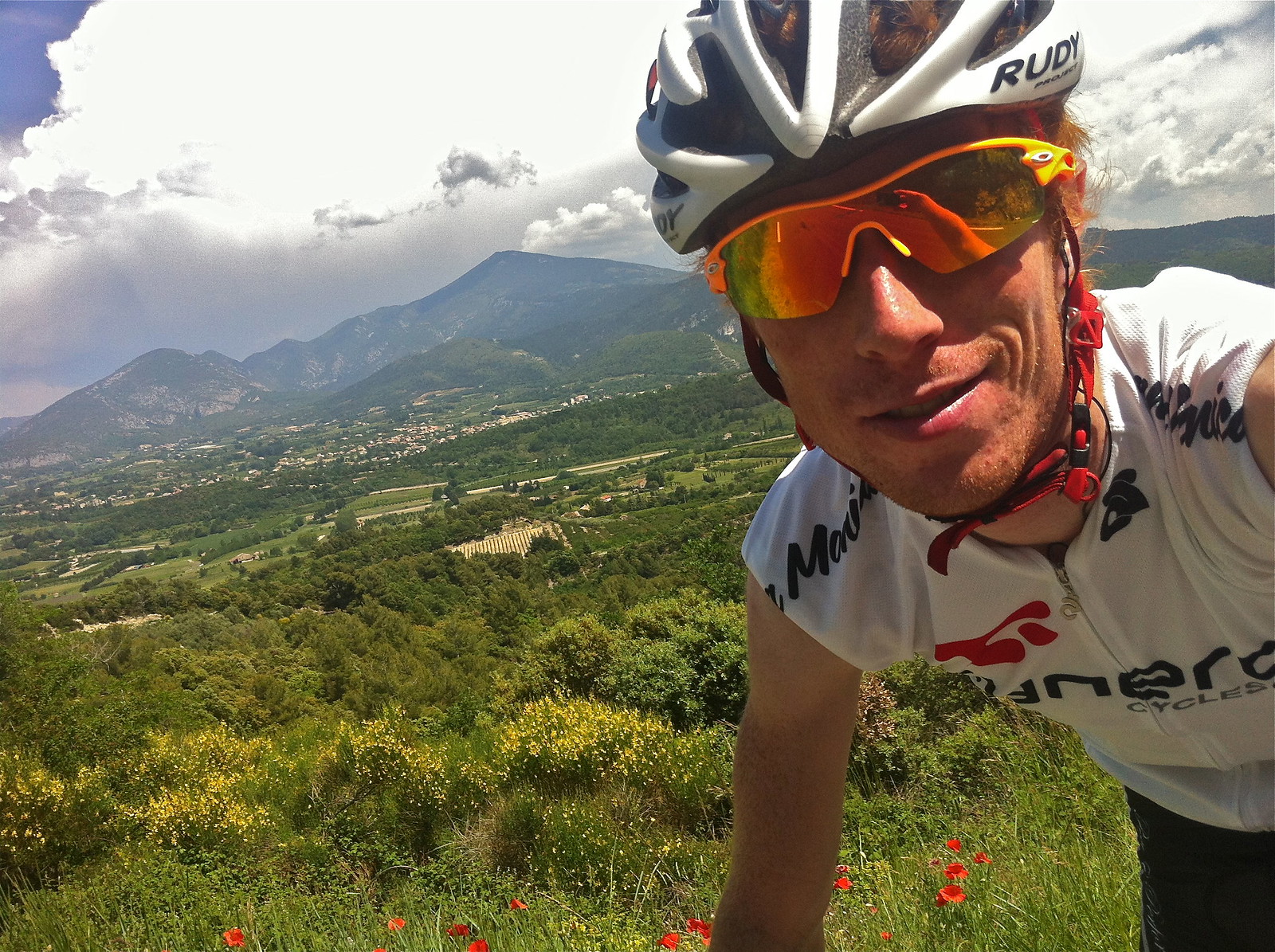The image captures a male mountain biker leaning forward on his bike, situated on the right side of the frame. He is smiling and wearing a white, sleeveless jersey adorned with black letters and a red logo. His attire includes black shorts and a distinctive white bicycle helmet trimmed in black, prominently featuring the brand name "Rudy" on the right side. The helmet's red strap is fastened securely under his chin. His sunglasses are highly reflective, showcasing orange and yellow hues, and you can glimpse the road reflected in them.

The background offers a stunning and expansive green landscape filled with fields, shrubs, greenery, pine trees, and scattered red flowers. In the far distance, at the base of a majestic mountain range, lies a small town or village. The mountains slope from the upper right to the lower center of the frame, encased by billowy white clouds and a sliver of blue sky, adding to the picturesque scenery.